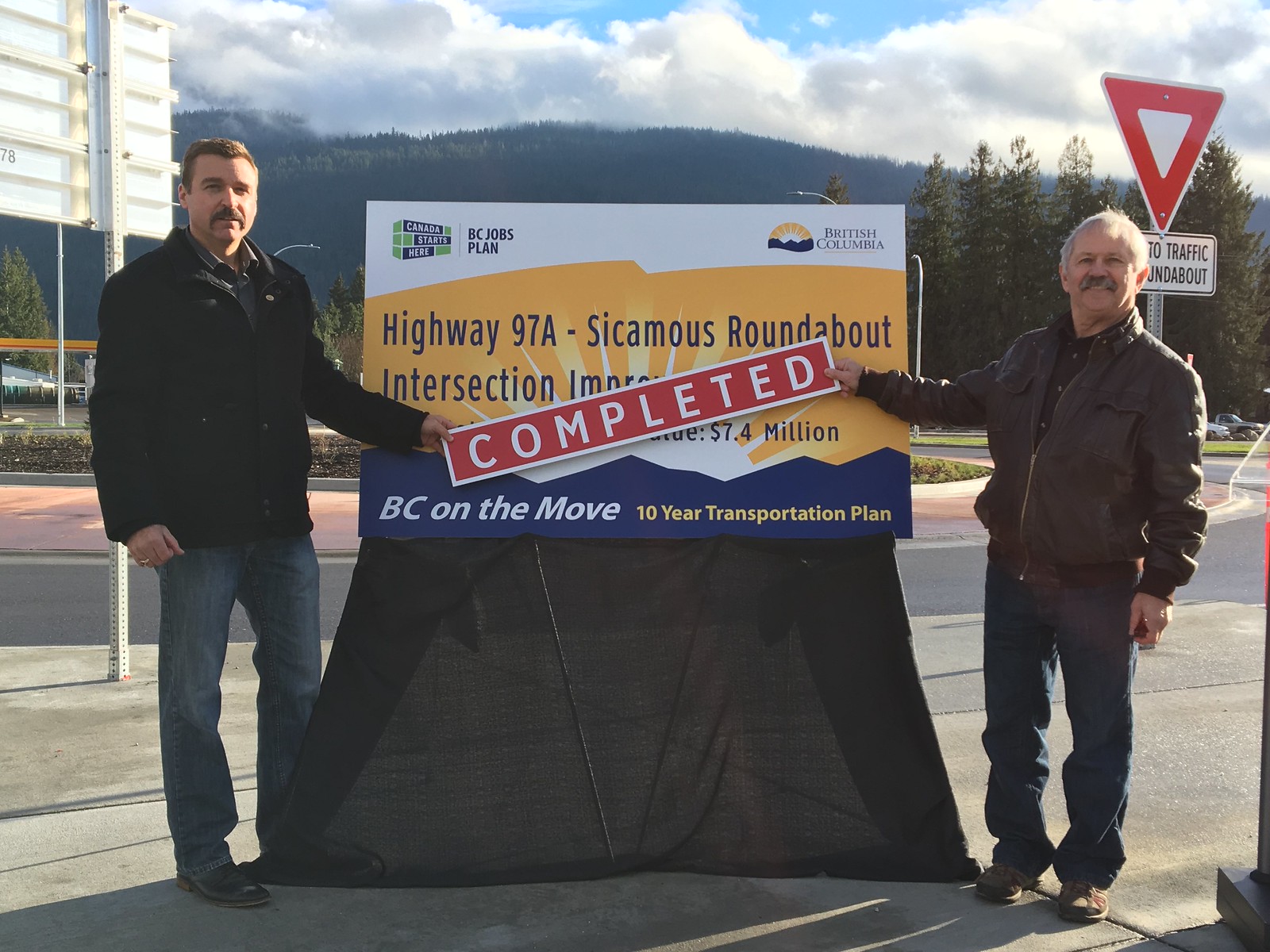In this picturesque setting featuring a vibrant blue sky dotted with puffy white clouds, two men stand on opposite sides of a sign on a sidewalk near a road, framed by a backdrop of tree-clad mountainous hills. The left side of the sign is flanked by a younger man sporting a dark mustache, short brown hair, a black jacket, and blue jeans. His counterpart on the right is an older, shorter gentleman with gray hair and a gray mustache, clad in a brown leather jacket, a blue button-down shirt, blue jeans, and brown tennis shoes. Both men hold rectangular boards reading "Completed" in red and white, partially obscuring the central sign. The primary sign reads "Highway 97A, Sycamus Roundabout Intersection," and beneath that, it declares "BC on the Move 10-Year Transportation Plan" in blue, yellow, and white lettering. This photograph celebrates the culmination of a significant $7.4 million project under the BC Jobs Plan.